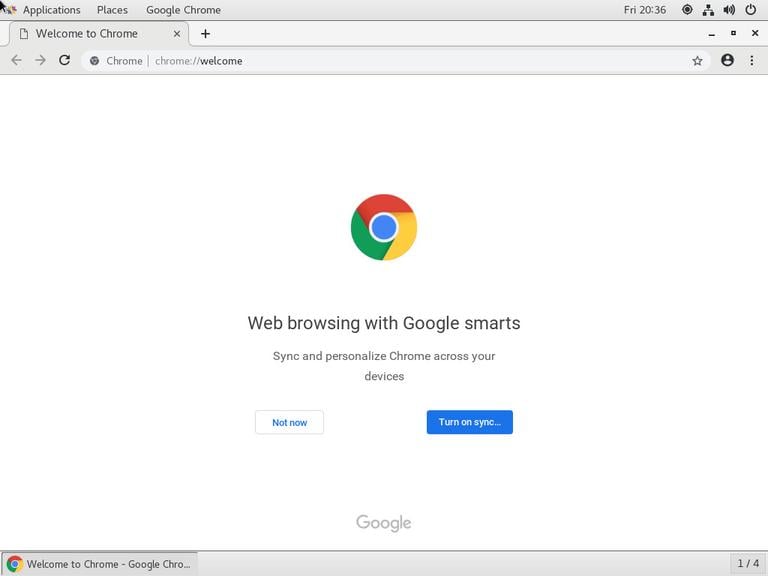This image is a detailed screenshot from Google Chrome, displaying the "Welcome to Chrome" tab. At the very top, there is a light grey banner featuring options such as "Applications," "Places," and "Google Chrome," along with the text "Friday 2036" on the right side. Various action icons are also visible in this top section. 

On the left side of the screen, there's a single browser tab open, titled "Welcome to Chrome." Directly beneath this tab is the web address bar, currently showing "chrome://welcome." 

The primary background of the page is completely white, prominently featuring the Chrome logo—a circular emblem with a blue dot in the center, surrounded by sections of red, yellow, and green. Below the logo, in black font, are the words "Web browsing with Google smarts." Following this is a line that reads, "Sync and personalize Chrome across your devices."

Two button options are provided beneath this text: "Not now" and "Turn on sync." At the very bottom, there's a greyed-out Google logo, and directly above it, another banner states "Welcome to Chrome, Google Chrome." This banner indicates it is one of four available panels.